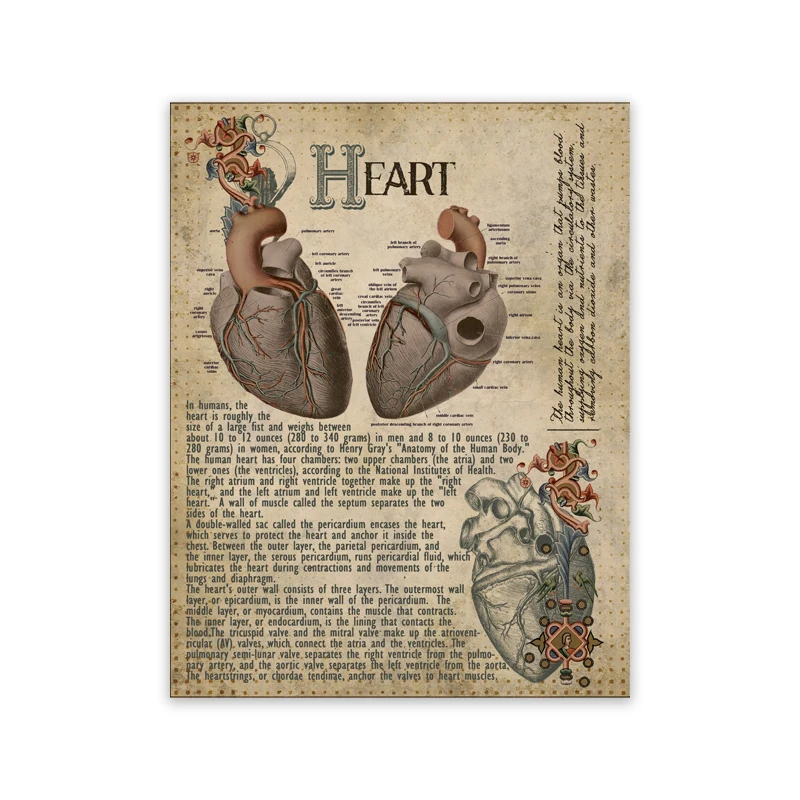This image depicts a detailed and informational page from an old, faded book, focusing on the anatomy of the human heart. Centrally, the word "Heart" is prominently displayed above intricate diagrams of the heart, which are labeled meticulously and show various views, including major arteries and veins. Additionally, handwritten cursive text runs vertically along the right side of the page, adding to the vintage feel. Below the diagrams, an extensive paragraph provides information from Henry Gray's "Anatomy of the Human Body," noting that in humans, the heart is roughly the size of a large fist and weighs between 10 to 12 ounces (280 to 340 grams) in men and 8 to 10 ounces (230 to 280 grams) in women. The text explains that the heart comprises four chambers: the two upper atria and two lower ventricles. The right atrium and right ventricle form the right heart, while the left atrium and left ventricle constitute the left heart, separated by a muscle wall known as the septum. The heart is encased in a double-walled sac called the pericardium, which protects and anchors it in the chest. Pericardial fluid between the layers of the pericardium lubricates the heart during contractions and movements. The heart’s outer wall consists of three layers: the outer epicardium, the middle myocardium containing the contracting muscle, and the inner endocardium lining. The tricuspid and mitral valves, known as the atrioventricular (AV) valves, connect the atria and ventricles, while the pulmonary and aortic valves regulate blood flow between the heart and the pulmonary artery and aorta, respectively. Cordae tendineae, or heartstrings, anchor the valves to the heart muscles.